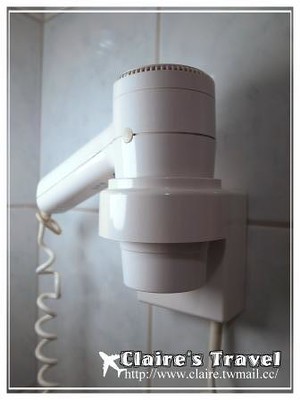The image showcases a close-up of a white, standard-sized hairdryer, commonly found in hotel bathrooms, securely affixed to a grey-tiled wall. The compact hairdryer, featuring a cylindrical body and a long handle, resides within a square-shaped wall holster designed specifically for it. The holster has a circular opening at the top, enabling the hairdryer to hang effortlessly. Attached to the hairdryer is a white, spiraled cord that descends downwards before looping back up to connect with the holster. The hairdryer's front and back sections are joined by a white nut. Below the hairdryer, in the bottom right corner of the photo, there is a label that reads "Claire's Travel," accompanied by the website "www.claire.twmail.cc" and a clipart-style icon of a plane.